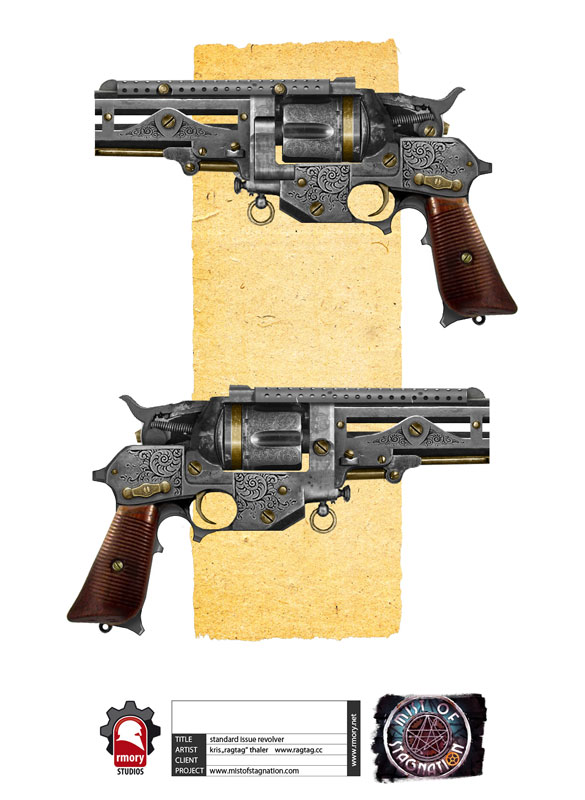The image features a vertically rectangular composition with a tan swatch of cloth serving as the background. Centered in the foreground are two intricately designed, steampunk-style revolvers, which appear to be the focal point of the artwork. The revolvers, with their ornate engravings and elaborate wooden handles adorned with golden rivets, are symmetrically arranged, facing opposite directions—one pointing left and the other right. Each revolver is crafted with a dual-layered barrel, featuring a hollow section between the upper and lower parts, and is embellished with an intricately designed heat guard with holes cut out of it. 

Additional detailing includes an intricate pattern around the trigger guard and sunlight-like carvings near the handle and the trigger. At the bottom left of the image, a logo with a red background resembling gears is visible with the text "Armory" beneath it. Adjacent to it, on the right, is a black square that contains the text "Mist of Stagnation." Below the revolvers, additional text provides more details: "RMORY Studios www.rmory.net Title Artist Client Project Standard Issue Revolver." This detailed composition evokes a blend of Old Western and steampunk aesthetics, reminiscent of weaponry from a video game.